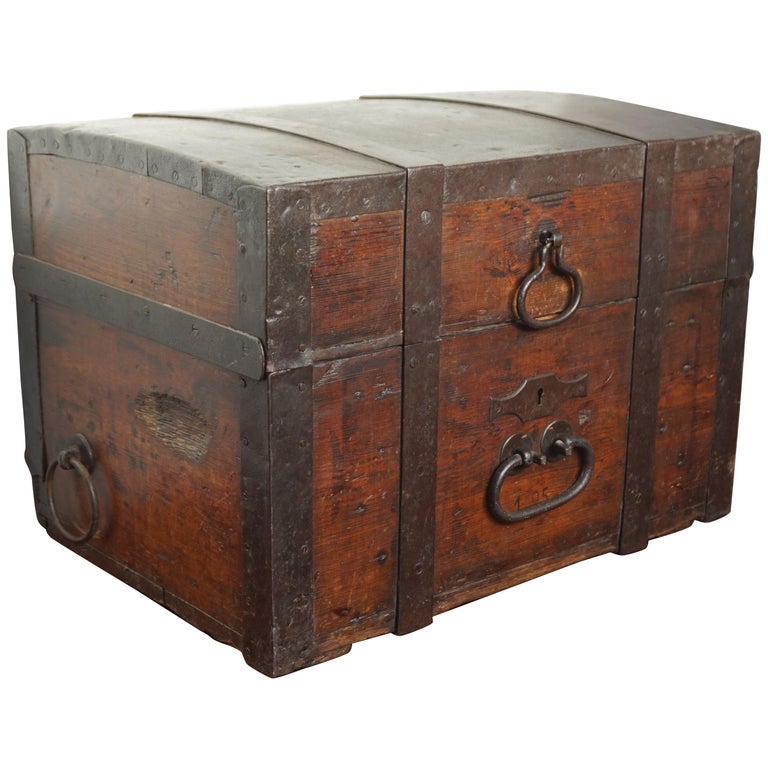The image showcases an antique wooden trunk positioned against a completely white background, displaying both a front and right-side view. The trunk is crafted from rich dark brown wood, framed and reinforced with matching dark brown metal borders and rods. It features two distinctive black metal handles on the front: a large oval-shaped handle at the bottom and a teardrop-shaped handle positioned above it. Between these handles, there is a visible keyhole, also made of metal. The right side of the trunk includes a circular metal ring handle situated at the lower left corner, suggesting it is used for carrying. The trunk's design includes a curved top, yet it maintains the overall shape of a horizontal rectangular prism. Despite its age and signs of wear with dents and marks, the trunk remains intact, exuding an antique charm.